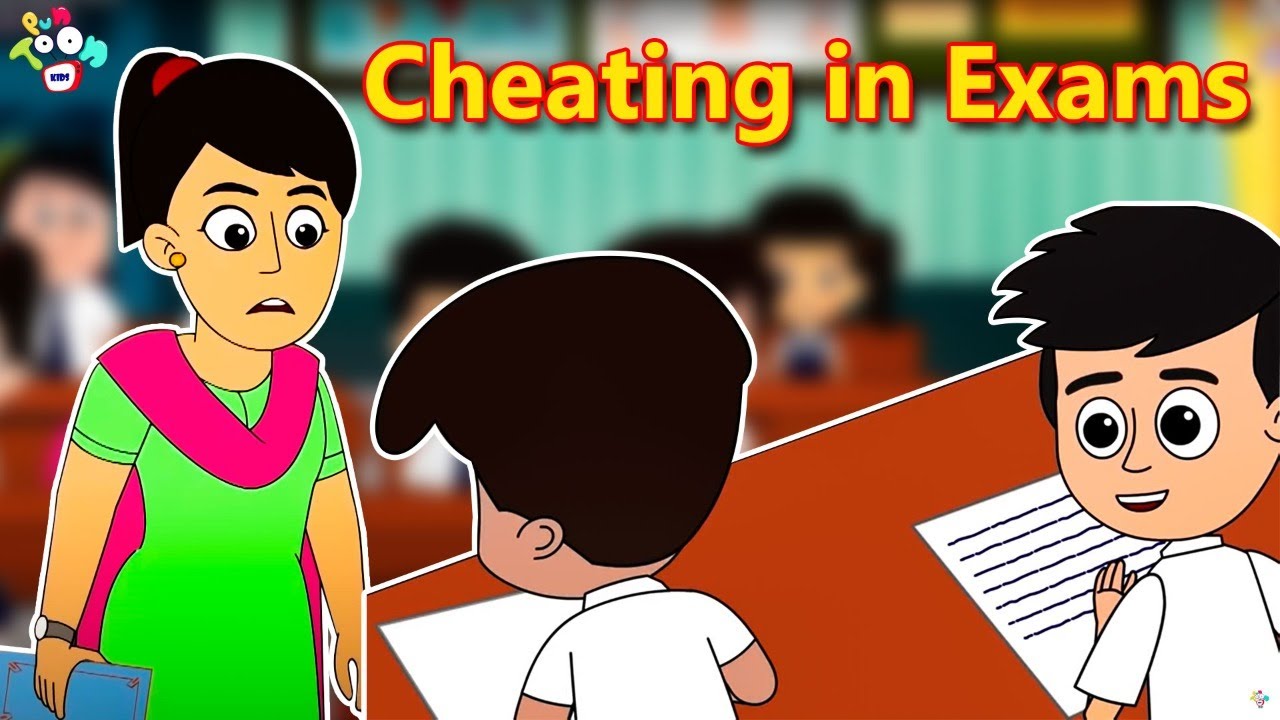The image, likely a scene from a cartoon or illustration by PUN Tune Kids, features the text "Cheating in Exams" in yellow letters outlined in red at the top right. In the top left corner, the PUN Tune Kids logo displays in a colorful mix of yellow, turquoise, pink, green, white, and blue against a red and white TV screen. Central to the image is a woman who appears to be a teacher. She looks upset, with her mouth turned downward, and is dressed in a bright neon green dress with a magenta scarf around her neck falling behind her. Her black hair is tied back in a ponytail with a red holder, and she wears a watch while carrying a blue folder. In the bottom right of the image, two students with black hair are seated at a brown desk covered with white papers, each dressed in white shirts. One student looks towards the teacher and the other at their peer, suggesting a potential act of cheating.